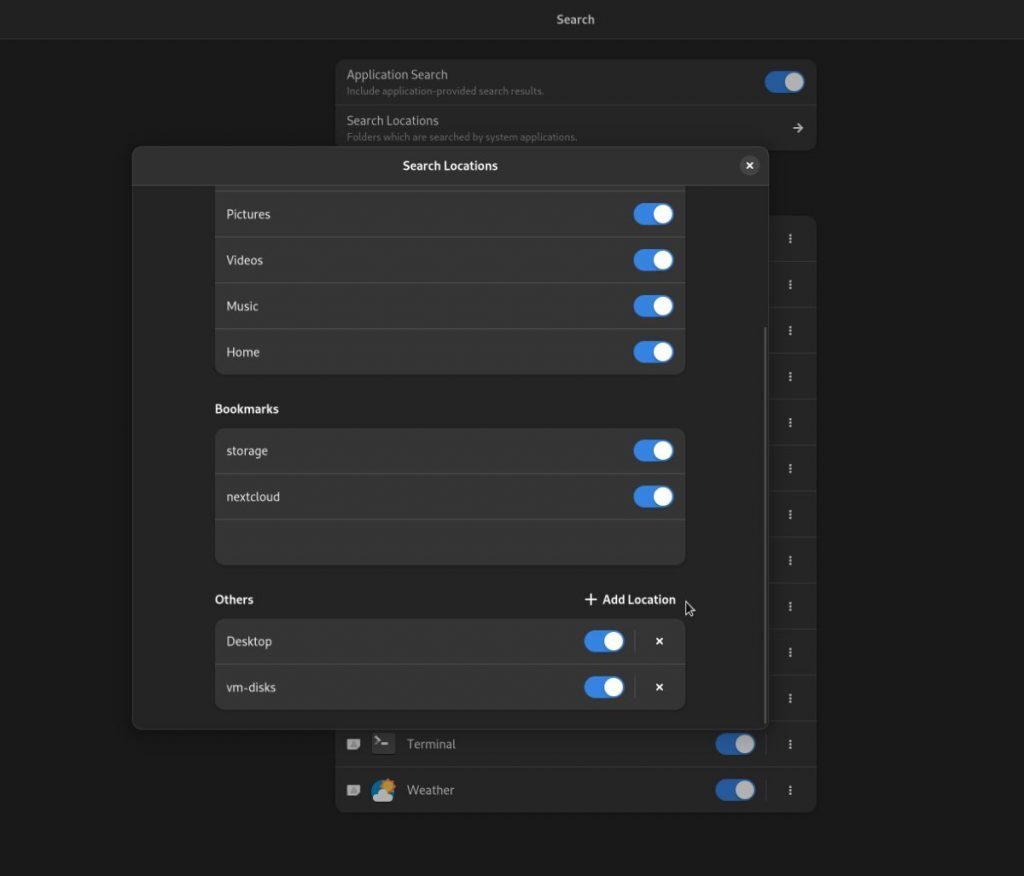The image features a user interface with a black background. At the top of the interface, there is a "Search" label. Below this, a gray box is titled "Application Search," which includes an application-provided search results option. To the right of this title is a blue toggle bar, currently switched on.

Underneath, the text reads "Search location folders which are searched by the system application." A small arrow pointing to the right is located on the far right side of this section. Below, a pop-up window labeled "Search Locations" appears, featuring a gray box with four lines, each representing a different category: "Pictures," "Videos," "Music," and "Home." Each category has a blue toggle bar to the right, all of which are switched on.

Moving further down, the section labeled "Bookmark" presents another gray box with two blue toggle bars, labeled "Storage" and "Next Cloud," both turned on. Finally, the "Others" section contains a gray box with two more blue toggle bars on the right side, corresponding to "Desktop" and "VM-disk" options on the left.